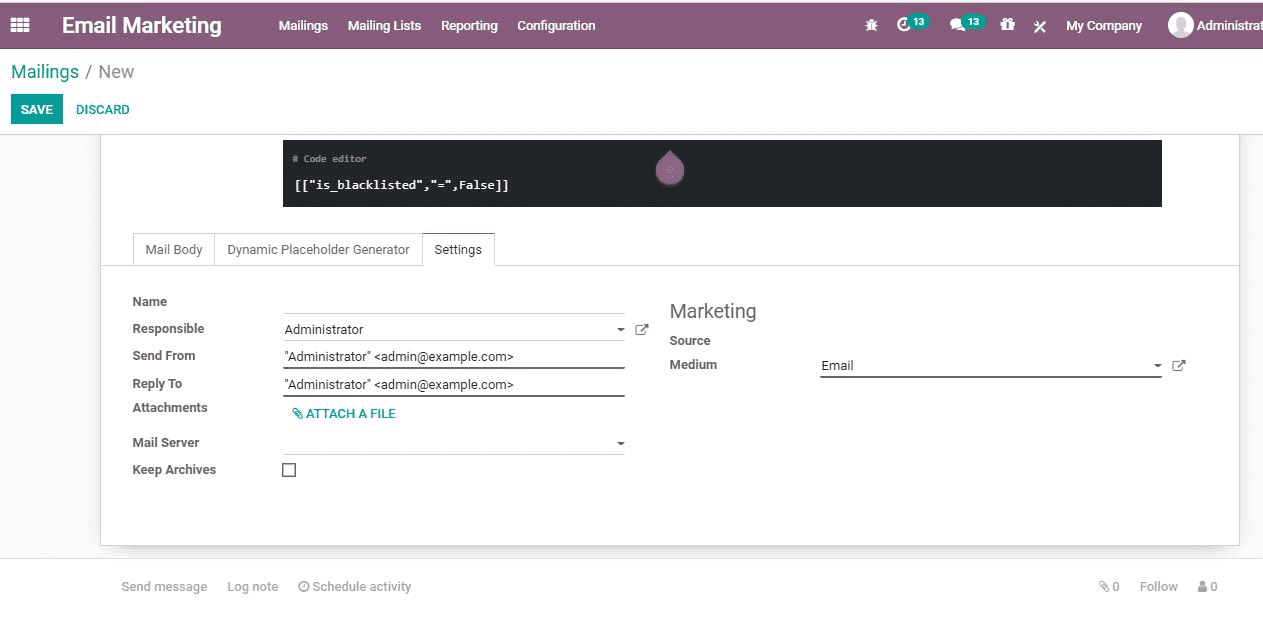This detailed image screenshot showcases an advanced email marketing dashboard. At the forefront, it highlights various functionalities including 'Email Marketing,' 'Mailings,' 'Mailing List,' 'Reporting,' and 'Configuration.' The interface appears to manage a total of 13 mailings, tagged under 'My Company' and 'Administration' categories.

Within the email composition area, it supports HTML for body content creation and dynamic placeholders for personalized email generation. Key fields include 'Name,' 'Responsible Sender,' 'Form,' and 'Server.' 

The user interface is equipped with a 'Code Editor' and options for 'Source,' 'Medium,' as well as tools to 'Attach File,' 'Send Message,' 'Log Note,' 'Check Activity,' and 'Follow' emails. Other available actions are 'Discard,' 'Save,' and navigate through 'Mailings' to oversee the campaign management effectively. This all-encompassing email marketing tool is designed to streamline the entire process, from drafting to sending and tracking emails.